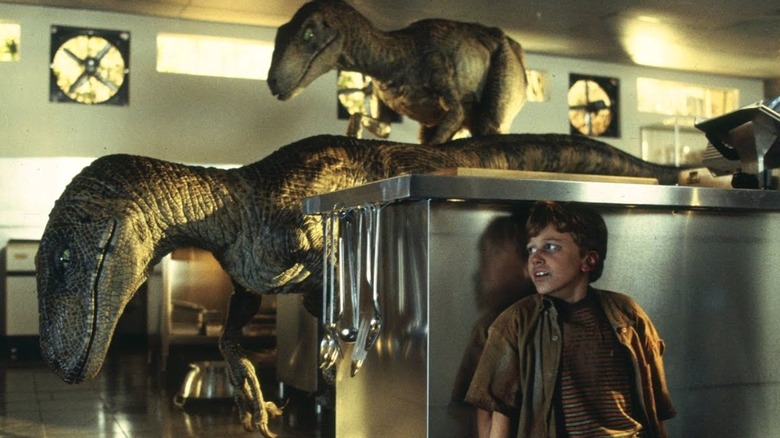The image appears to be a still from a movie, likely one of the Jurassic Park films, showing a high-tension scene set in a kitchen environment. A terrified young boy, dressed in a dirty brown and striped shirt, is hiding beneath a stainless steel kitchen table. His disheveled appearance suggests he's been running and hiding, possibly through mud. Suspense builds as two dinosaurs, characterized by dark brown and gray scales with olive green eyes, search for him. One dinosaur, with sharp claws and a long mouth, is perilously close, standing on a kitchen table, while the other prowls behind another table. The kitchen itself is detailed with gray walls, three black-slatted extractor fans near the ceiling, and horizontal windows lining the upper half of the walls. The shiny tiled floor reflects a few more stainless steel tables in the background, and a set of serving spoons hangs from the end of the table where the boy is concealed.